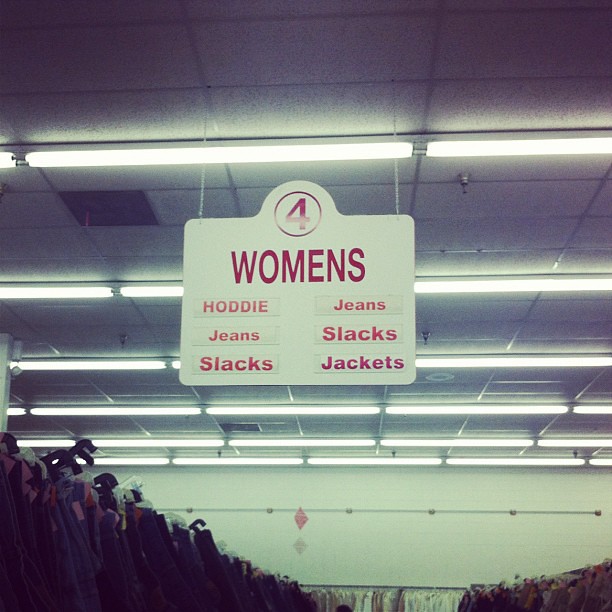A white ceiling sign inside a store, photographed from floor level, hangs by two chains. The sign, labeled with the number "4" in bold red to indicate the aisle, features additional text in dark red: "Women's" followed by a list of items. "Hoodie" is misspelled as "Hoddie," along with "Jeans" and "Slacks" on one side, and "Jeans," "Slacks," and "Jackets" on the other. The ceiling is lined with long fluorescent lights and office tiles. Below the sign, rows of clothing racks extend on both sides, and a shopper's head is visible. The rear wall of the store is white.